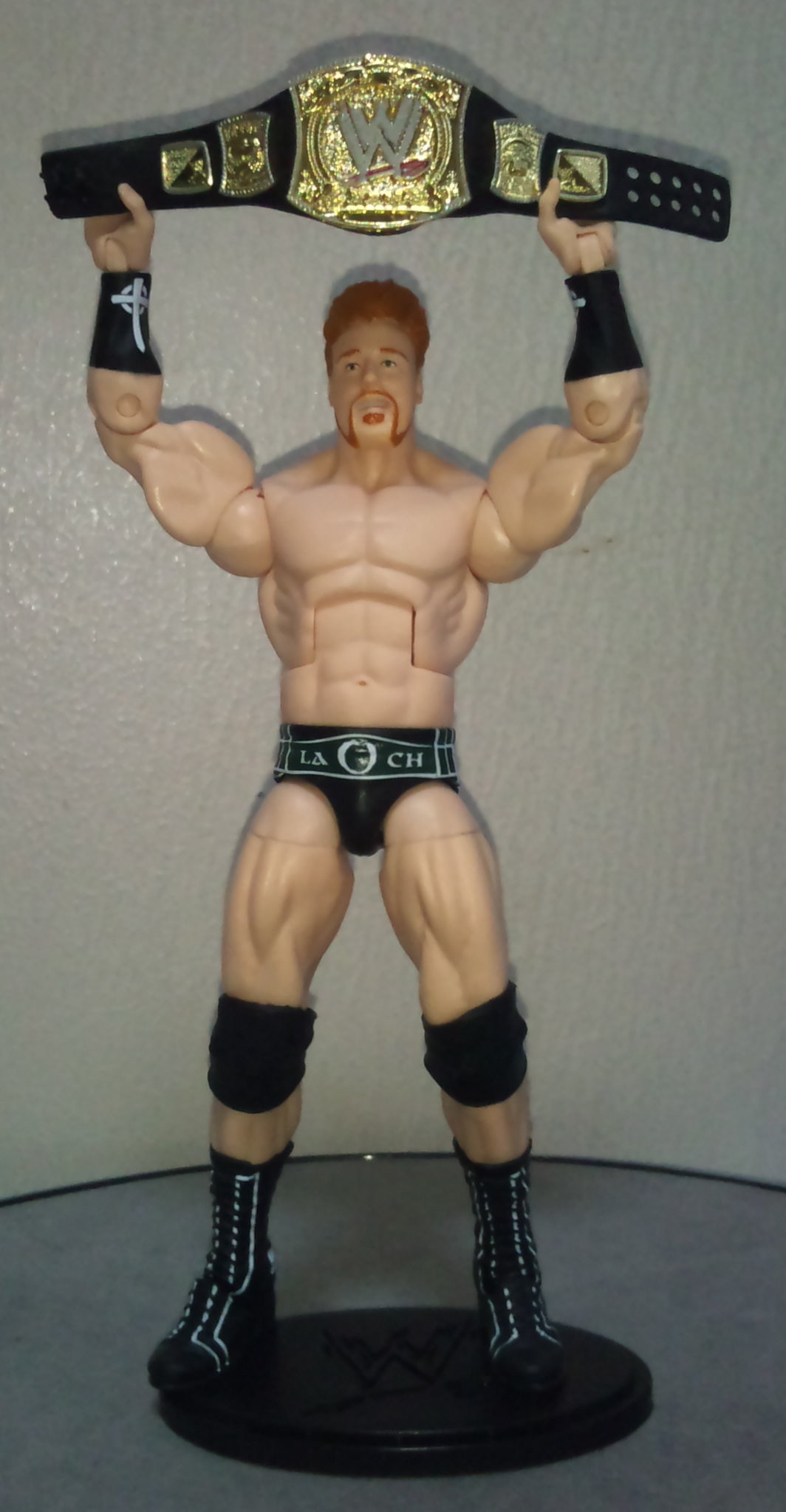This photograph showcases a highly detailed action figure of a professional wrestler, prominently displayed against a white painted wall and situated on a round table. The action figure is mounted on a small, black plastic circular base and is posed with arms raised, holding a large, ostentatious championship wrestling belt above its head. The belt is black, adorned with multiple gold symbols, a prominent gold buckle, and a silver "W" in the center, indicating its status as a WWE championship belt.

The wrestler, depicted as a muscular white male with orange hair and beard, is outfitted in classic wrestling gear. His ensemble includes black wrestling boots with black laces and white stripes running down the sides, black knee pads, and black wristbands, one of which is detailed with a cross. The figure is clad in tight black Speedos that feature the letters "LA" and "CH" in opposing corners. These intricate details, combined with the figure's stance and accessories, capture the dynamic and competitive spirit of professional wrestling, making it an impressive collectible.